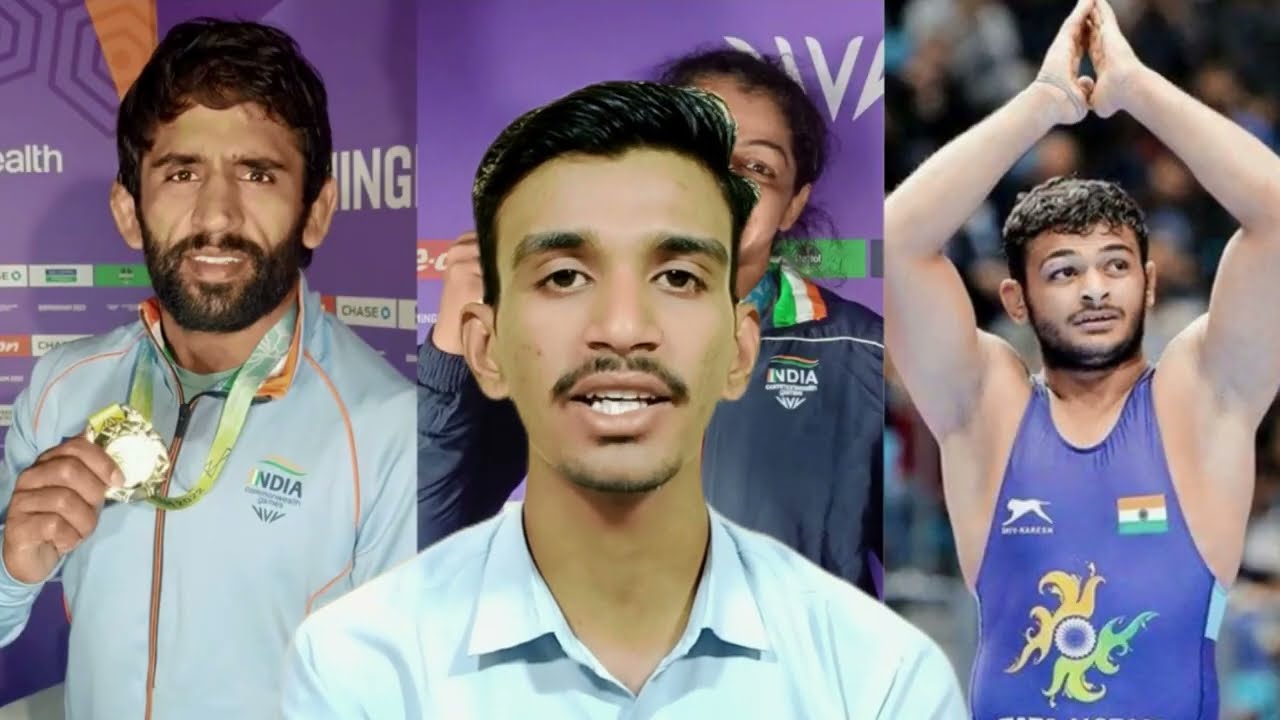This composite image features a central close-up of an Indian man with slicked-back dark hair wearing a blue collared shirt, seemingly speaking or presenting. Behind him are three side-by-side photographs highlighting different Indian athletes, likely from the Olympic Games. On the left, a bearded man with a short beard is dressed in a light blue jacket, holding a gold medal with a ribbon around his neck. The middle photograph contains a man wearing a blue track jacket, partially obscured by the shadowy eyes of a woman behind him. The right photo shows another bearded man in a purple wrestling suit adorned with the Indian flag emblem, his hands raised in a victorious triangular pose. The backgrounds of the left and middle photos are purple, creating a cohesive visual theme. This collage collectively celebrates Indian athletes and their accomplishments in sports.